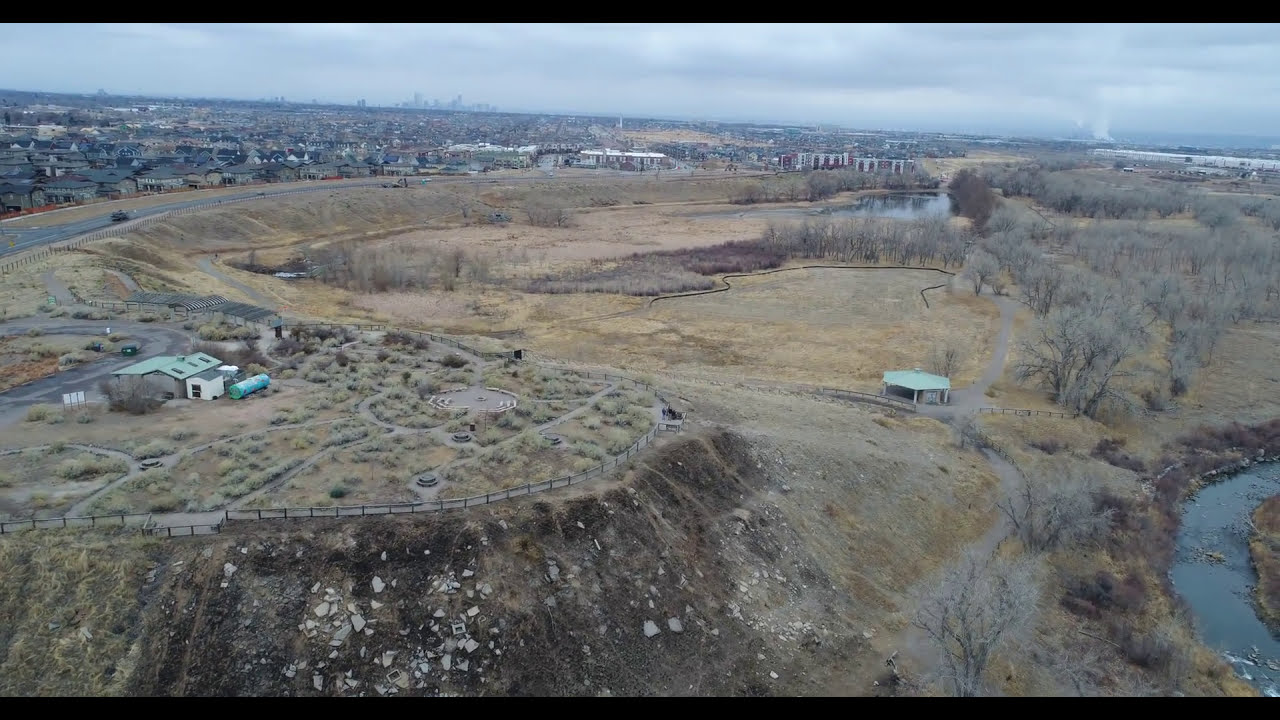In this image of an expansive outdoor landscape, an open field dominates the lower three-fourths of the frame, covered in lightly brown and tan hues suggestive of late fall. Sparse patches of green are visible amidst the mostly dead and brown trees that flank the field. To the right, a small, tranquil river meanders through the scene, while a light green-roofed gazebo stands prominently nearby. To the far left of the open field lies a storage area characterized by structures with light green roofs and a possible turquoise propane tank. Embedded within this field, a cement structure, likely a helicopter landing pad, is also discernible.

In the upper portion of the image, notably in the top eighth, a dull, overcast gray sky looms, casting a subdued light over the landscape. Just below the sky, the horizon is lined with gray-roofed houses extending in a seemingly endless row, transitioning into larger buildings and possibly a cityscape in the far background. The leftmost part of the upper quarter features a more densely built area, contrasting with the sparse placement of structures in the open field below. Despite the mix of natural and man-made elements, the overall composition of the image lends itself to a quiet, somewhat desolate atmosphere typical of a late autumn day in a park or an undeveloped tract of land.